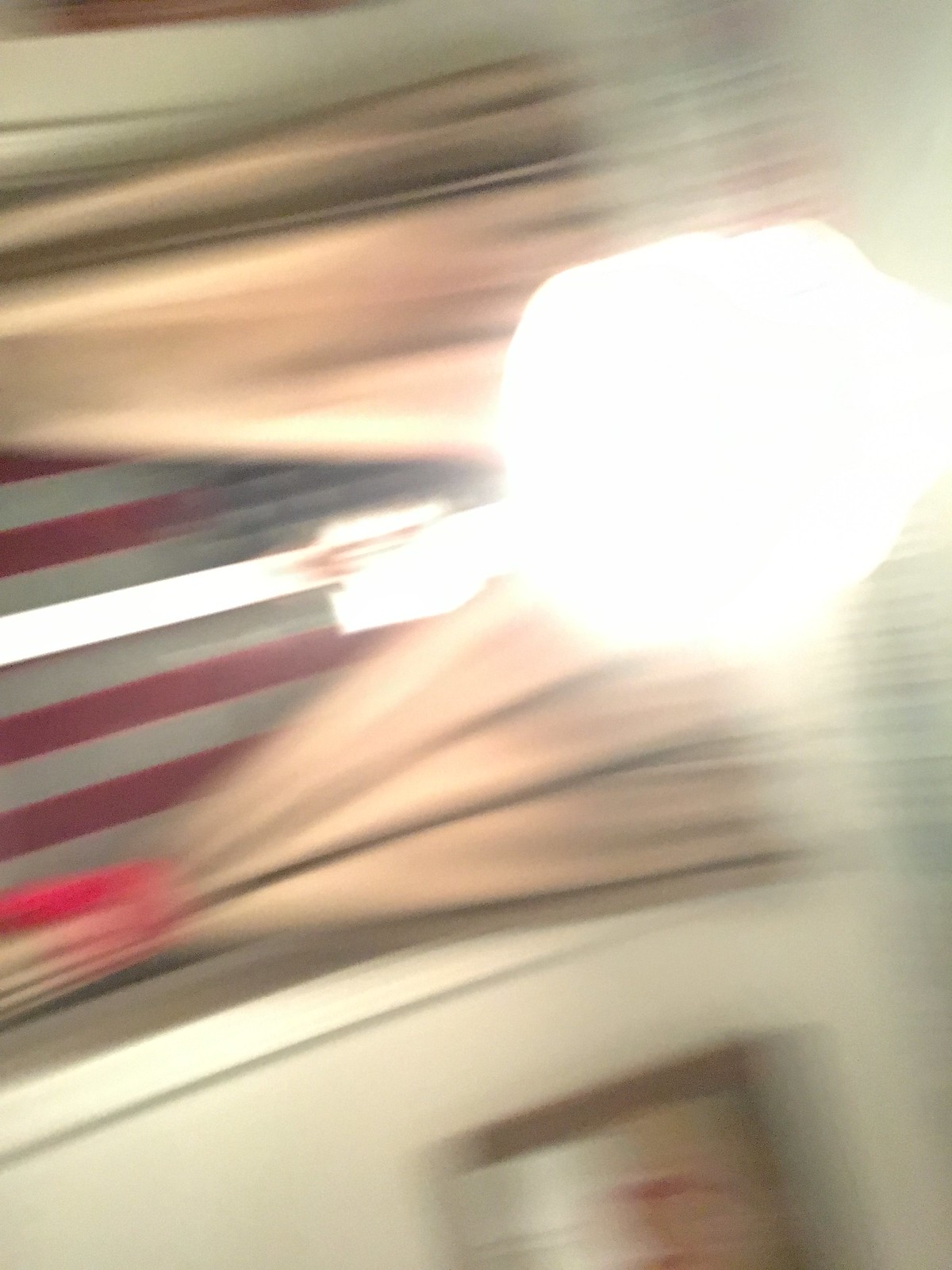The photograph appears to be taken indoors, capturing a room in significant motion, resulting in a highly blurry image. Dominating the right-hand side is a large, glowing orb with bright, intense yellow and white light radiating outward, contributing to visible orange-tinged motion lines. Above and slightly to the left of this light source, there is a window with a curtain draped on the left, revealing the reversed stripes and partial stars of an American flag through the blurry lens. Below the blurred window area, there's a red smudge that could be interpreted as a fire extinguisher against a cream-colored wall. Additionally, on the bottom left of the image, a portion of a picture frame hangs on the same wall. All elements are surrounded by a backdrop of primarily white, and the fabric near the middle is tied with a red tie, adding to the chaotic visual effect.